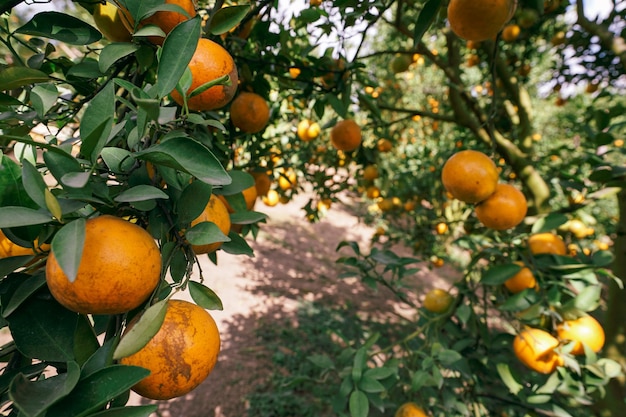This vivid image captures a thriving orange orchard brimming with lush, ripe fruit ready for harvest. The robust trees are laden with healthy, vibrant oranges, their branches sagging under the sheer weight of the bounty. Sunlight streams through the verdant canopy, creating dappled patterns of light and shadow on the ground below. Interestingly, the photograph is taken from an elevated perspective, offering a unique view that showcases the expansive orchard, including the healthy, evenly shaped trees and the sunlit earth beneath them. The fruit, about the size of a baseball, looks incredibly inviting and could easily tempt anyone to reach for a fresh orange. The scene is a visual feast, hinting at the labor and care invested in maintaining such a thriving garden, and perfectly capturing the essence of harvest time in this picturesque grove.